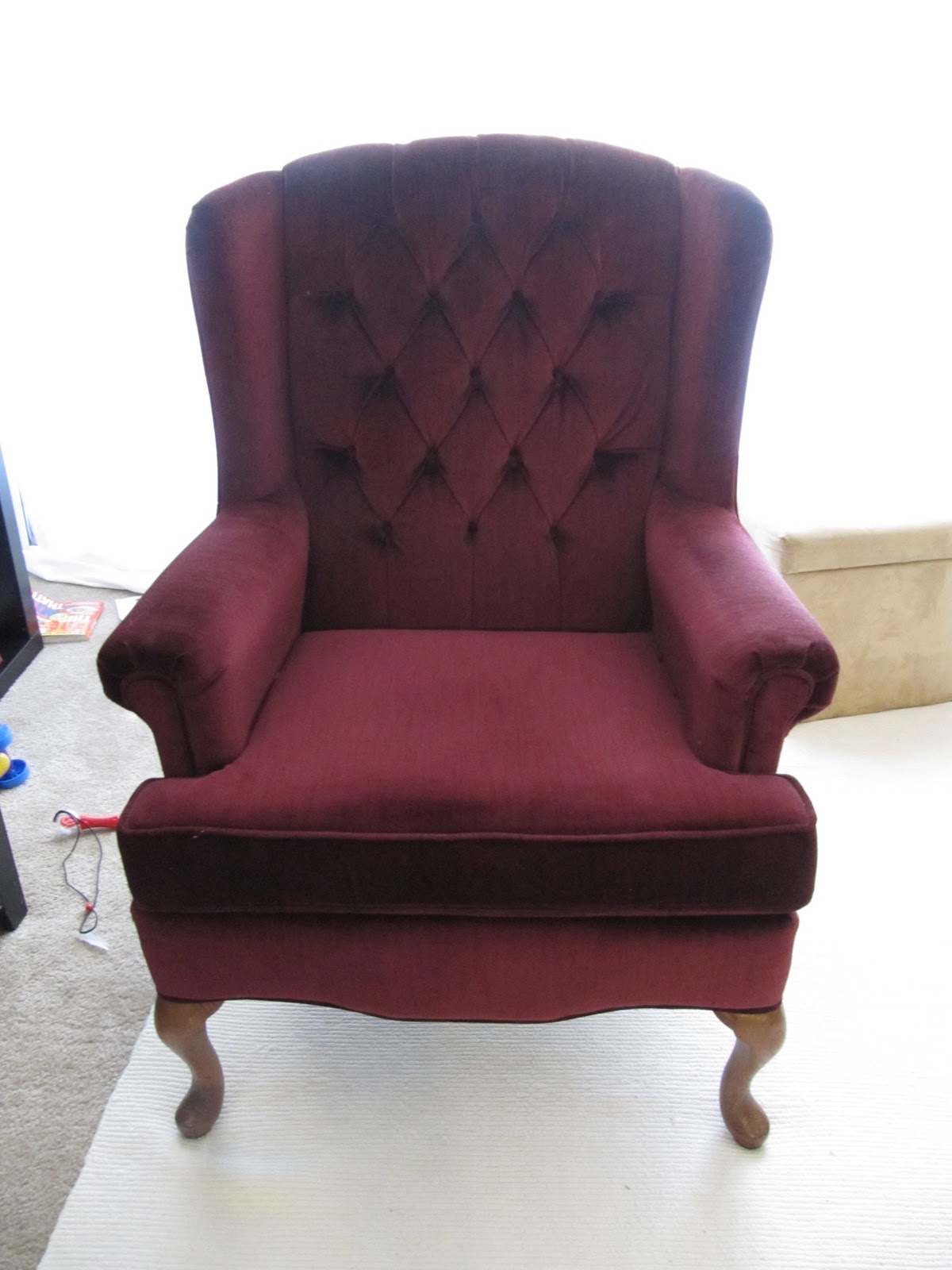This photograph captures an intricately detailed scene of an old-style Victorian armchair placed at the center of a brightly lit room, showcasing a blend of elegance and comfort. The high-backed sitting chair, with its deep oxblood or burgundy velvet upholstery, features a quilted button-tuck design, enhancing its classic appearance. The well-crafted wooden legs are curved and finished in a rich brown, adding to the chair's vintage charm. Resting on a white rug, the chair serves as the focal point amid a scattering of objects. To the right, a beige square object, possibly an ottoman or chest, is partially visible. The background hints at a modern living room setting, with glimpses of a gray carpet, magazines, toys, a red object possibly resembling a flute, and a mesh tie on the floor. A window or door in the image allows bright light to flood the scene, highlighting the details and colors that include shades of blue, red, and beige. Overall, the photograph presents a serene yet intriguing room filled with subtle details that invite closer inspection.